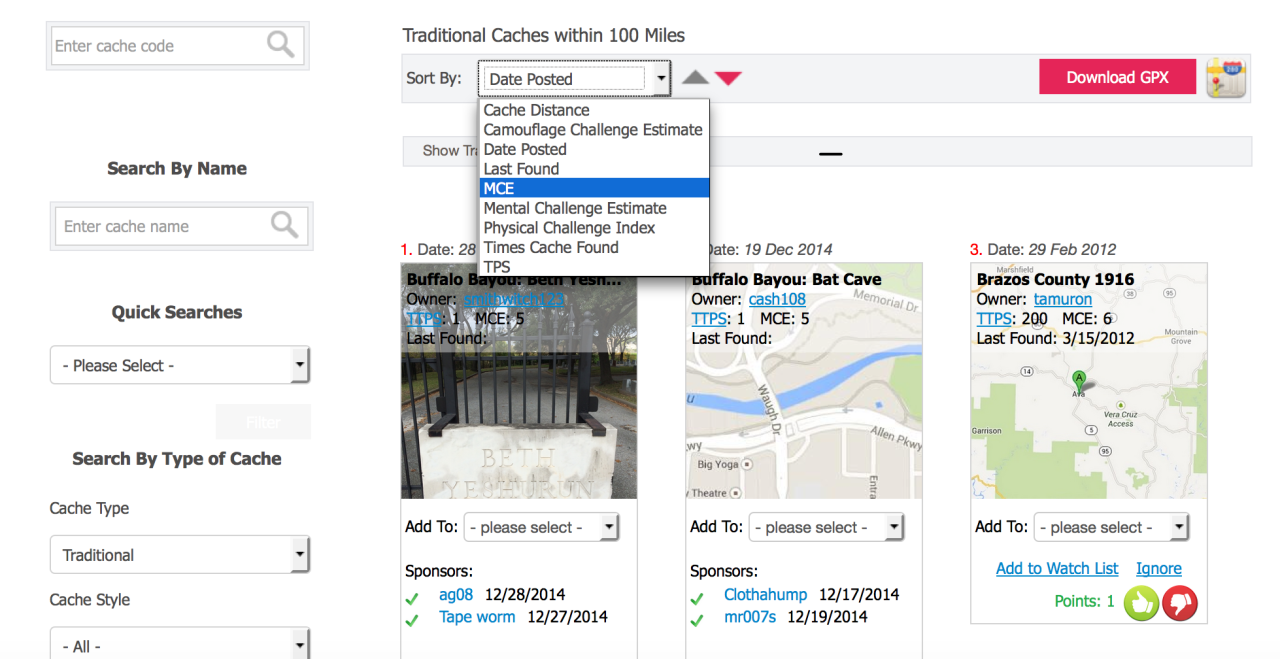At the top left of the image, there's a search query field bordered by a thick light gray outer border and a medium gray inner border that reads "Enter Cache Code" in a muted tone. Adjacent to this field on the right, there is a gray magnifying glass icon. Below this, in bold black text, it reads "Search by Name," followed by another search field labeled "Enter Cache Name," also accompanied by a gray magnifying glass icon to the right.

Further down, the text "Quick Searches" is also highlighted in bold black. Directly beneath this, there's a drop-down menu. The menu indicates the option to "Please Select," with a downward-facing arrow in a tall rectangular light gray area, flanked by dashes on each side. Just below to the right, there's a faded gray icon resembling a filter; this appears to be disabled until a selection is made from the quick search options.

Continuing lower, the text "Search by Type of Cache" is prominently bold in black. Under this heading, it presents two drop-down menus—one labeled "Cache Type" showing "Traditional," and another labeled "Cache Style" displaying "- All -".

At the top right, it states "Traditional Caches within 100 miles" in a summarized format. Beside this, there is a sort option labeled "Sort by," with an open drop-down menu showing "MCE" in capital letters as the selected option. To the immediate right of the sort menu, a rectangular red button displays "DOWNLOAD GPX" in capitalized white text. 

Adjacent to this, to the far right, a map is visually represented within a bubble-like icon.